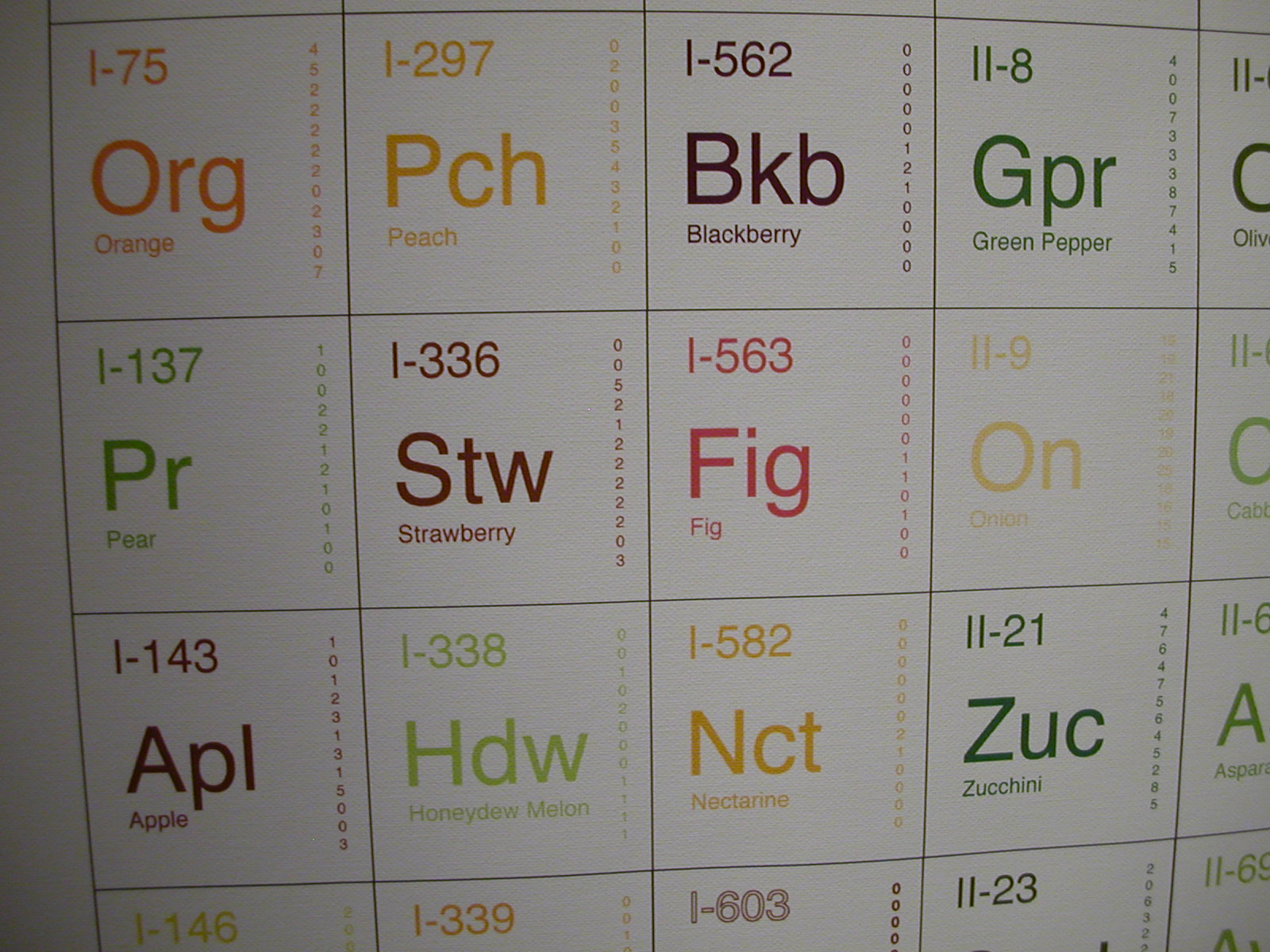This image features a creatively designed chart mimicking a periodic table, but instead of chemical elements, it displays various fruits and vegetables. Each item is enclosed within a black-bordered square and is organized in rows from top left to right. The entries include details such as an identification number, a three-letter abbreviation, and the name of the fruit or vegetable. For instance, one square reads "I-7-5-O-R-G" in orange font, indicating "orange," while another square reads "I-2-9-7-P-C-H" in yellow font for "peach." Additional entries include "I-5-6-2-B-K-B" in black for "blackberry," followed by listings for green pepper, pear, strawberry, fig, onion, apple, honeydew melon, nectarine, zucchini, and more. Each square's text color corresponds to the color of the respective fruit or vegetable. The chart is centrally positioned in the image, styled as a poster, and possibly serves as a visual aid or educational tool, though its precise purpose is unclear.